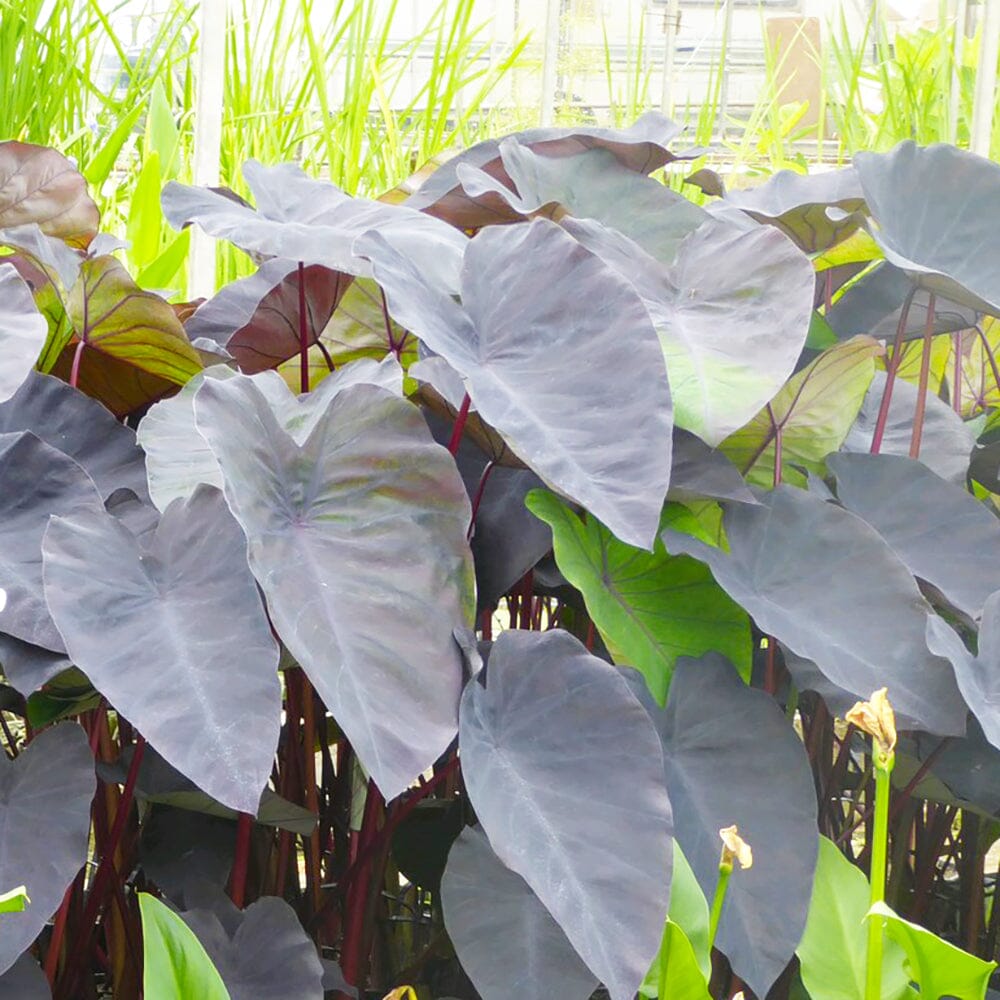This vibrant photograph showcases a lush scene of diverse plants thriving under the bright sun. Central to the image are heart-shaped leaves exhibiting a striking blend of colors: primarily grayish-tan with hints of green and brown, and prominent veins of purple. These leaves grow from sturdy red stems, adding a rich contrast to the foliage. Scattered among these are clusters of large, purple-tinged leaves, creating a vivid display against the intricate network of green leaves surrounding them. At the base of the plants, small flowers peek through, framed by green leaves. The background features tall, verdant grass-like shoots bathed in sunlight, adding depth and a serene backdrop to the close-up botanical beauty.